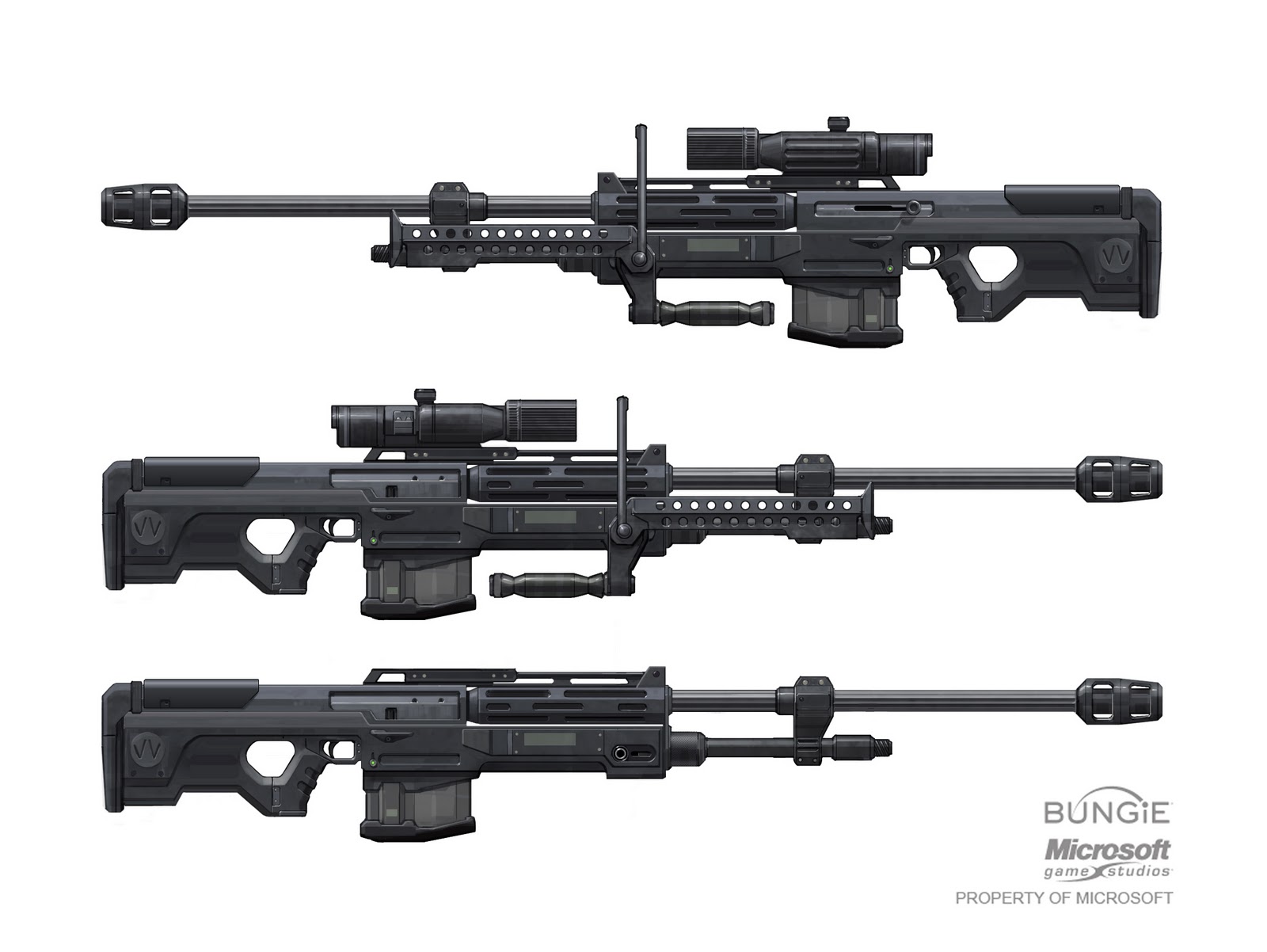This detailed illustration depicts three automatic military-style assault rifles from a video game or gaming guide, meticulously drawn in a realistic style. The rifles are stacked vertically; the top rifle faces left, while the two below face right. Notably, the bottom rifle differs slightly from the top two, missing some illustrative parts like a handle or guide, which are present on the others. In the lower right-hand corner, the image is marked with a logo stating "Bungie Microsoft Game Studios, property of Microsoft," suggesting it is sourced from Microsoft gaming content.